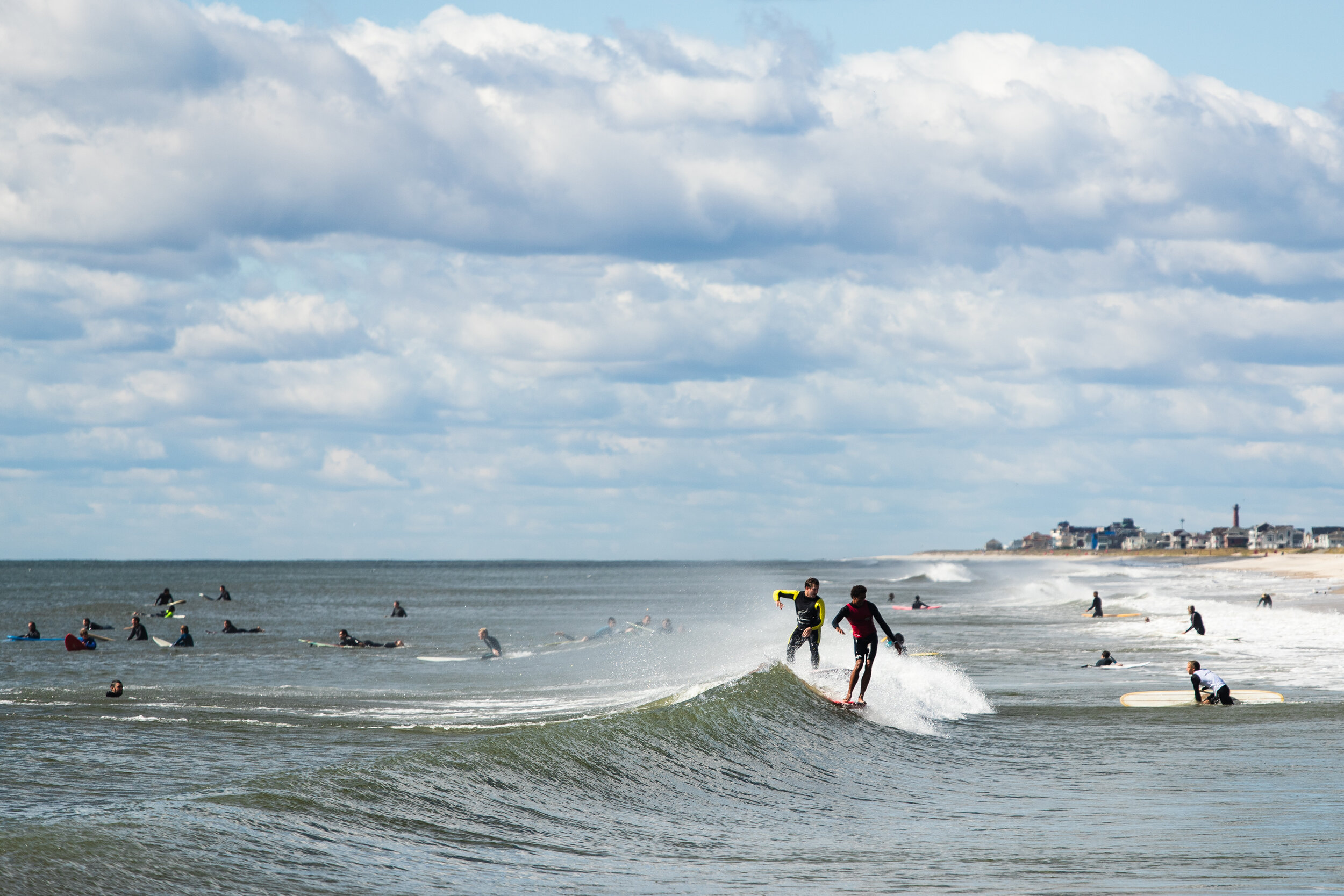This rectangular photograph captures a vibrant beach scene with various surfers populating the greenish ocean water near a coastline. Dominating the upper part of the image, the sky is a light blue canvassed with rows of white, fluffy clouds with darker undersides, but not appearing stormy. In the middle section, a wave crests with two surfers riding it; one is in a black wetsuit with yellow accents, positioned on the left, and the other is in a red and black wetsuit, positioned on the right. Around them, approximately 20 other surfers can be seen: about 12 to 13 on the left side and 7 to 8 on the right, either paddling or waiting for the next wave. In the distant background to the far right, a vague cityscape emerges with several buildings barely discernible. A sliver of sandy beach and some cottages are also visible near the center right of the image, adding a serene backdrop to the lively ocean scene. White foam from the breaking waves is scattered throughout, adding dynamic texture to the water.